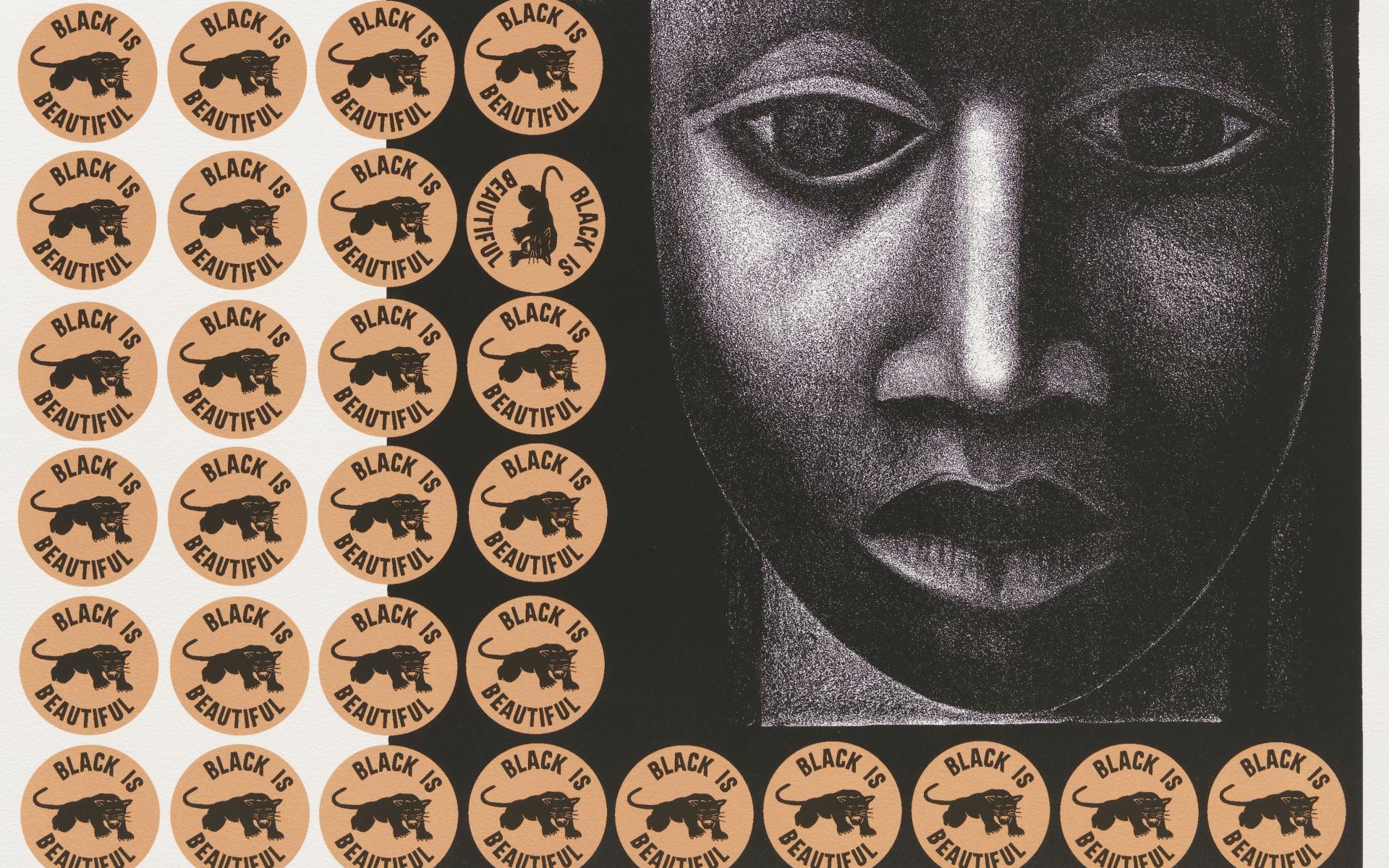The image is a composite artwork featuring a detailed drawing of an African American face with feminine features. The face, which resembles a wood-carved mask, has large, determined eyes, a pronounced nose, and full lips. This striking face occupies approximately 40% of the right side of the piece, set against a dark background. Surrounding the face, particularly to the left and bottom, is an array of 29 round, orange medallions arranged in a grid of four across and seven down, with an additional row at the bottom. Each medallion bears the phrase "Black is Beautiful" with a black panther depicted in the center. The background to the left of the face is white, contrasting with the darkened background on the right, emphasizing the face and medallions in the composition.